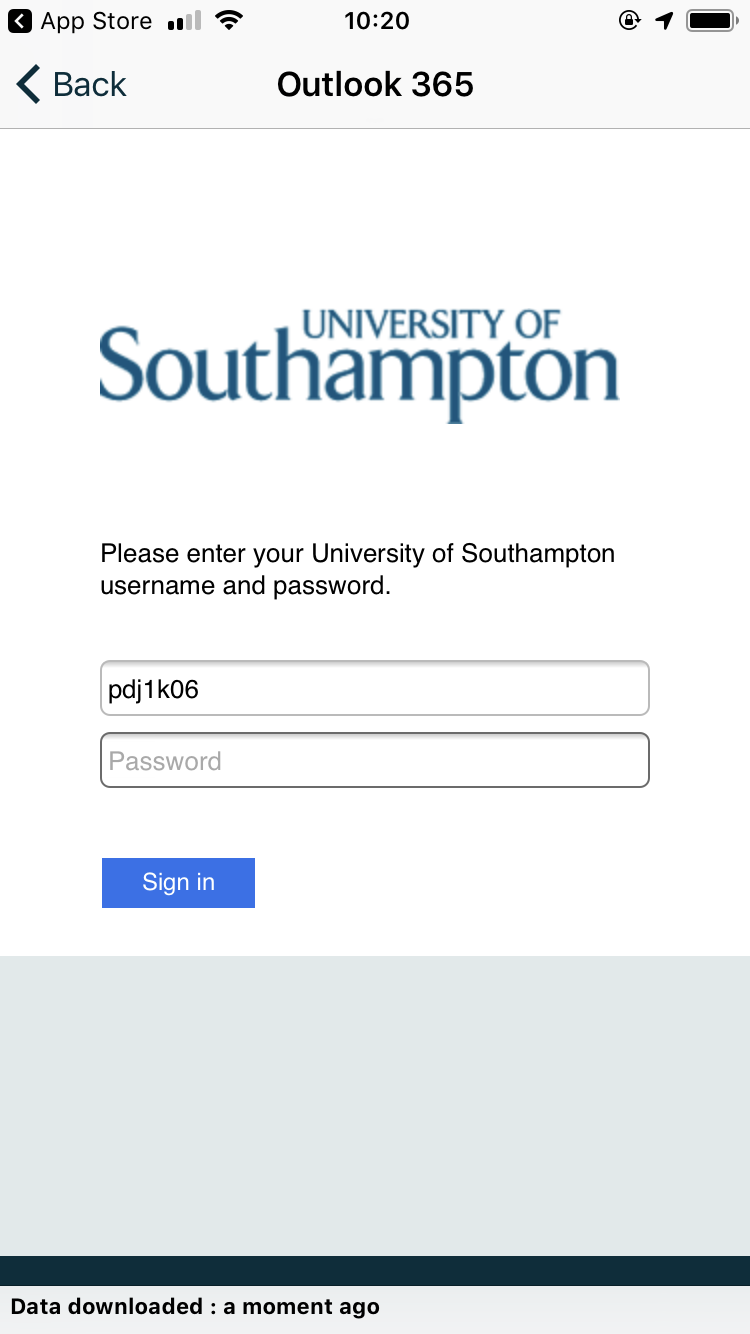Here's a cleaned-up and detailed caption for the image you described:

---

Screenshot of the App Store at 10:20 AM with a nearly full battery (99-100%). The title of the app page is "Outlook 365." On the main section of the page, with a white background and blue text, it reads "University of Southampton." Below that, in black text, it prompts users to "please enter your University of Southampton username and password." There are two input fields: The top field is labeled "Username" and is already filled with "pdj1k06." The bottom field, for the password, is empty but has a placeholder text in light gray indicating "password." Beneath the input fields, there is a blue "Sign in" button with white text. The bottom portion of the page features a large, light gray rectangle with a dark blue bar at the bottom. Below this bar, in black text, it notes "data downloaded a moment ago."

---